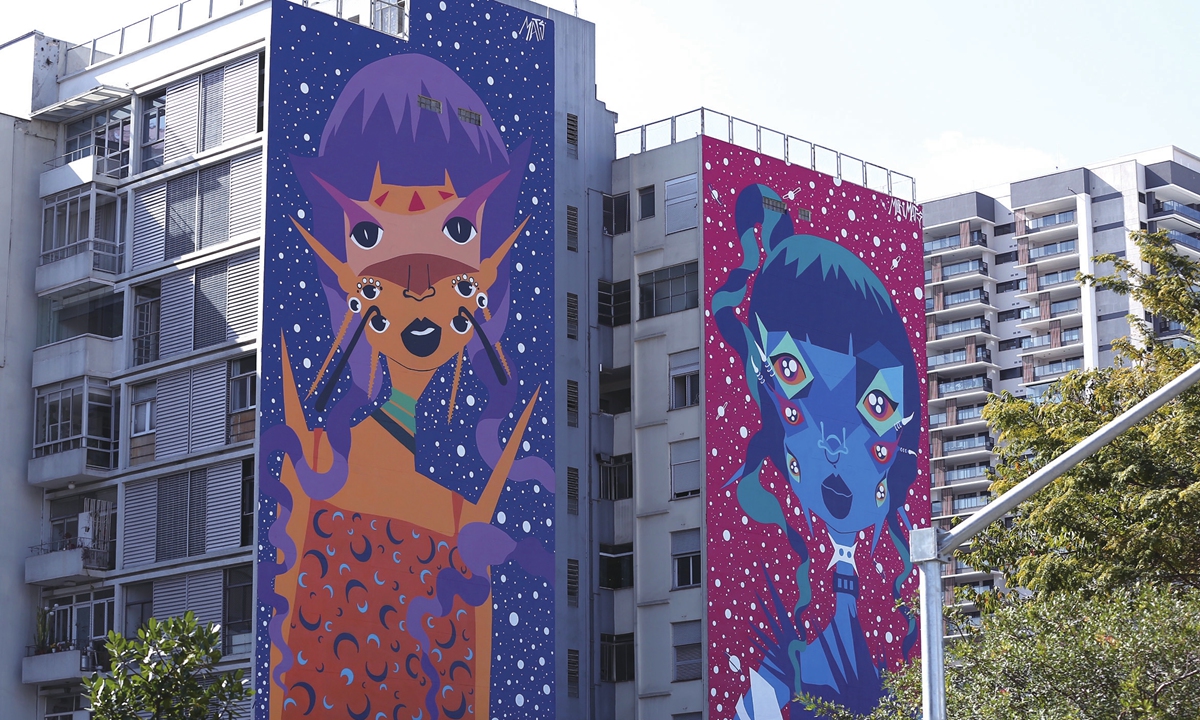This is an outdoor daytime photograph of multi-storied apartment buildings, at least seven stories high, with several taller buildings visible in the background. The buildings have balconies and bushes lining the sides, as well as a stairway. Prominently featured on the facades of these buildings are two sizable, surrealistic paintings that extend several stories high.

The painting on the left showcases a woman with blue hair, regular features like two eyes and a nose, but also has three additional eyes on each cheek. She wears a red dress adorned with dark and light blue moons and two blue ribbons and a black choker around her neck. The background is depicted with a blue and white space theme, featuring large and small white dots resembling stars.

The painting on the right features another fantastical woman with blue hair and multiple eyes arranged at the center of triangles on her cheeks. She has two noses and a star-shaped white symbol on her neck, along with a dark blue band marked with three slits. The background here is red with white planets, contributing to an overall cosmic and otherworldly aesthetic. Each painting is highly detailed, with intricate designs on the clothing and background, capturing a blend of surrealism and celestial motifs.